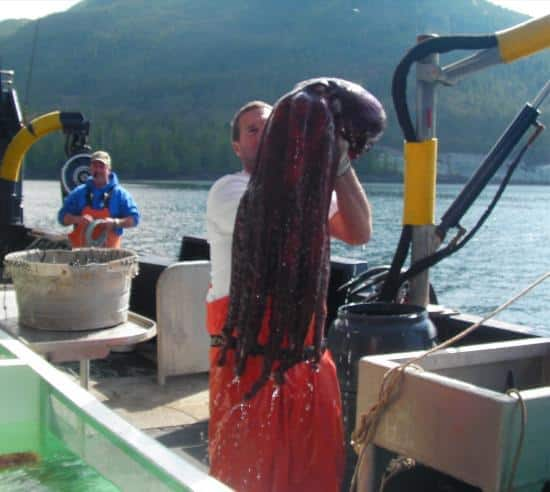The colored photograph captures a lively scene on a fishing boat, set against the backdrop of clear blue water and a distant, tree-covered hillside that stretches to the top of the frame. At the center, a man dressed in a white shirt and water-repellent red pants dominates the image, holding up a colossal, dripping black or brown squid that extends nearly as tall as he is. His face is obscured by the squid's sprawling tentacles. Light reflects off the squid and the liquid dripping from it, emphasizing the bright, sunny daytime conditions. 

Behind him, another man in similar fishing gear can be seen, wearing a blue shirt and an apron, engaged in activities typical of a fishing expedition. To the left, partially visible, is what seems to be a wooden tub or tank while on the right, the boat's equipment includes metal bars forming a framework and a tank for holding fish or other aquatic specimens. The left side of the image also features a long rod apparatus with yellow wrappings that extends out over the water, hinting at the fishing operations. The scene is bustling with activity, framed by a sliver of sky on the top left and right, giving a sense of the open, expansive outdoor setting.